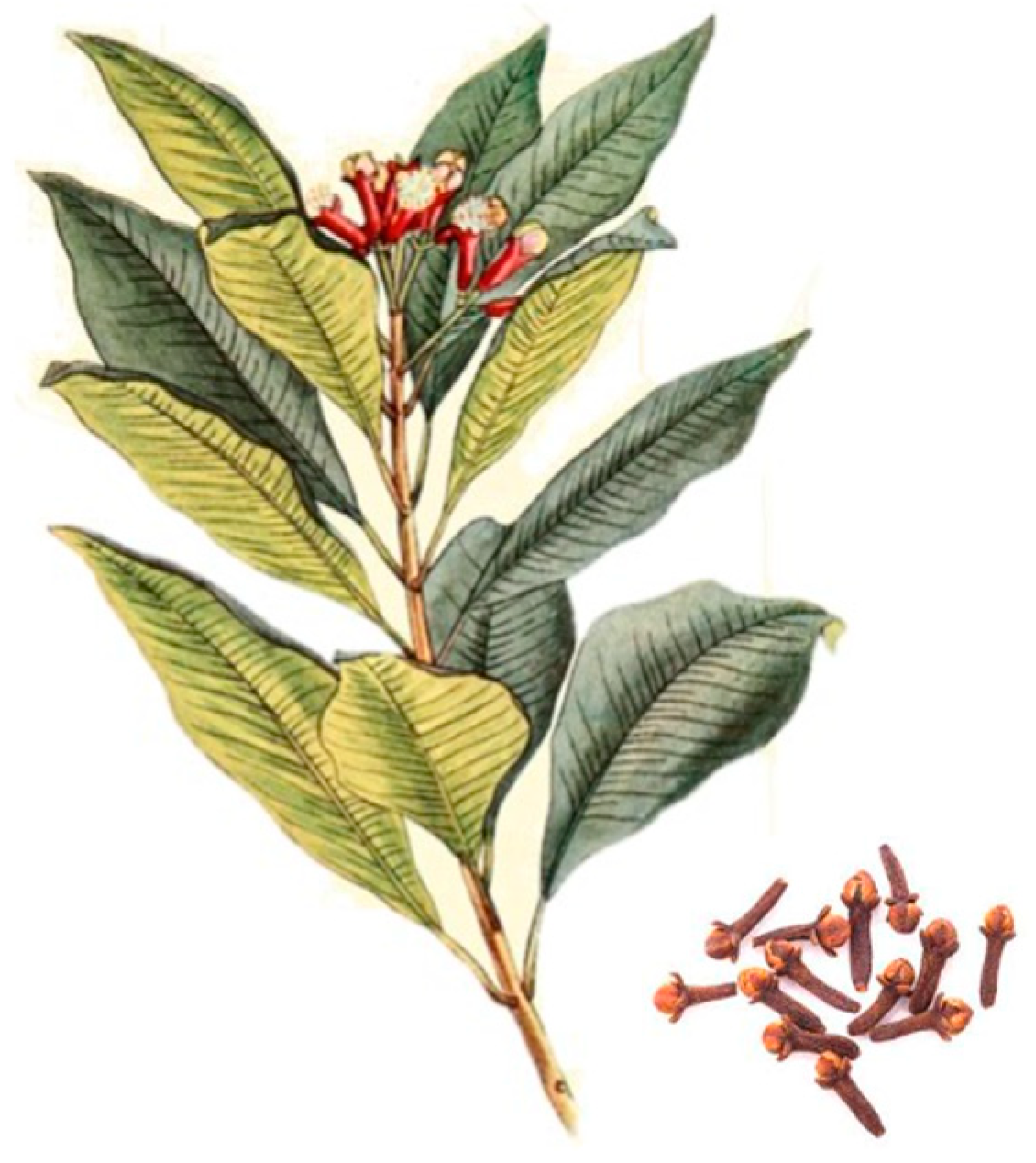This detailed image combines illustration and photography to present the clove plant. The drawing on the left side showcases the plant's structure: a brown stem with abundant dark and light green leaves. At the apex of the stem, clusters of reddish flowers with white tips, resembling honeysuckles, stand out. On the bottom right, a photograph displays the transformation—about a dozen dried clove seed pods are arranged in a circle. These seed pods are a mix of dark brown bodies and light brown tops, intricately connecting the botanical illustration to its harvested spice form.